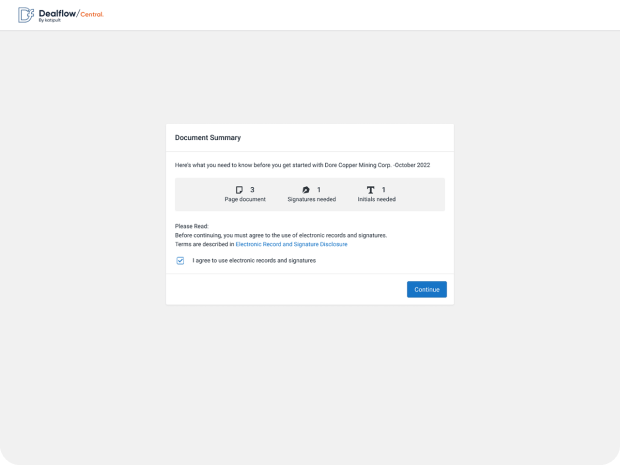The screen capture image features a user interface related to document processing. At the top of the screen, there is a blue logo with a stylized "D" and "F" on it, along with the text "DealFlow / Central" in a mix of black and orange colors.

Beneath this heading, a large gray box occupies the main portion of the image, centrally featuring a smaller white box. The white box contains text in various font colors: black, blue, and white. At the top, it prominently displays "Document Summary" in black font. Below this heading, black text reads, "Here's what you need to know before you get started with Dunn Copper Mining Group, October 2022."

Directly beneath this, a thin gray rectangle includes detailed document information: 
- "Three-page document" (with a small paper icon),
- "One signature needed" (with a small pen icon),
- "Initials needed: 1" (with a 'T' icon).

Further down, black text prompts the user: "Please read before continuing. You must agree to the use of electronic records and signature terms as described in Electronic Record and Signature Disclosure." The phrase "Electronic Record and Signature Disclosure" is highlighted in blue, indicating a clickable link.

At the bottom of the white box, there is a blue square box with a checkmark beside the statement in black, "I agree to use electronic records and signatures." The user is then provided with a call-to-action button: a blue rectangle with white font stating "Continue."